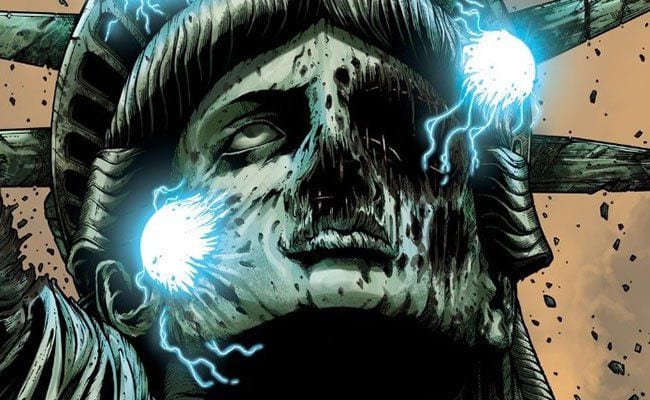The image is a detailed graphic art piece, reminiscent of comic book styles, focusing on the head of the Statue of Liberty being violently destroyed by bright blue electrical orbs. Only the face of the statue is depicted, with significant damage: its left eye socket and cheek are crumbling and hollow, the nose has been eroded away, and there are holes and black marks pocked across the green facade. Two prominent, glowing blue orbs, connected by tendrils of electricity, interact destructively with the statue—one attacking the right cheek and the other emerging from the left eye socket. The backdrop features a turbulent orange sky, resembling a dust-filled atmosphere, with bits of debris and stone rubble cascading from the statue's crown. The overall scene conveys an unnatural, chaotic force disintegrating this iconic symbol, set against a distressed, apocalyptic environment.